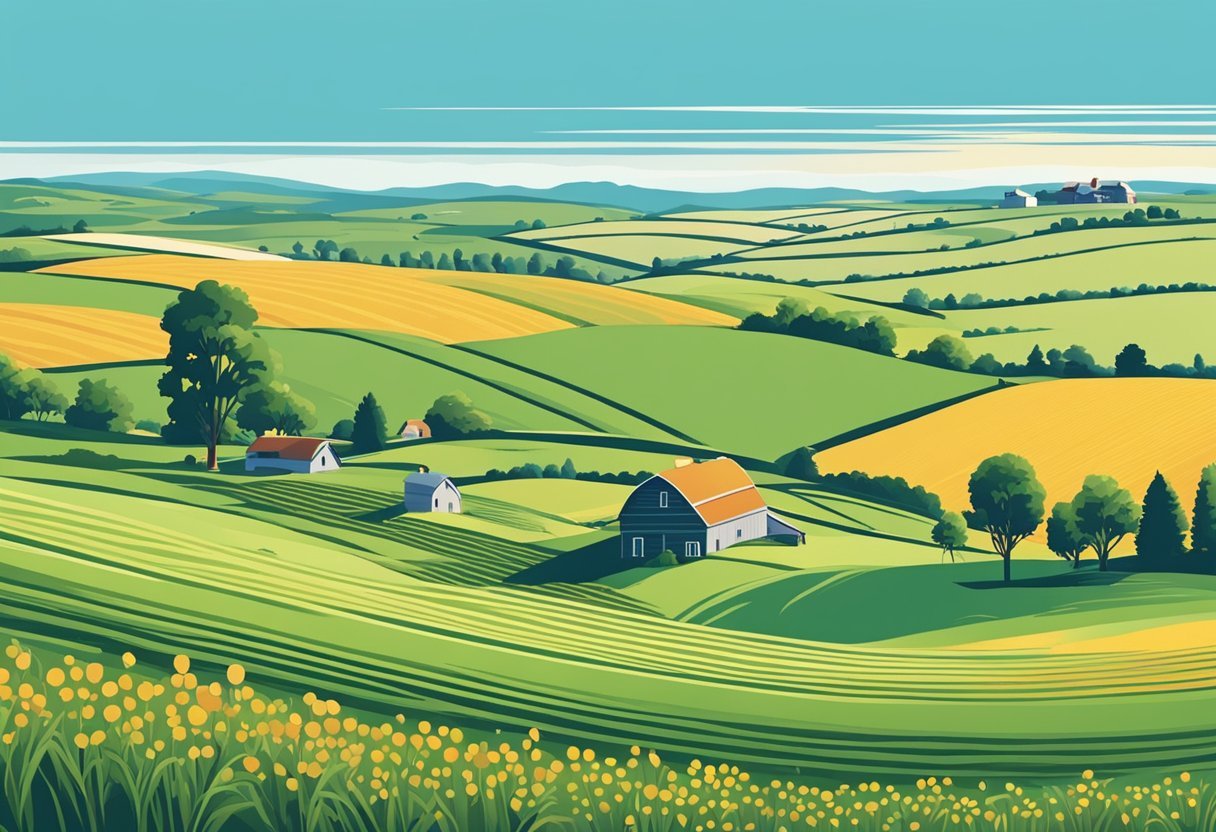This detailed digital artwork, likely AI-generated, portrays an expansive and picturesque farm landscape. In the immediate foreground, vibrant yellow wildflowers, possibly daffodils or daisies, add a touch of color. Rolling farmlands unfold behind them, featuring a farmhouse, a barn, and various outbuildings, with a few scattered trees providing a natural accent. The land is segmented into a patchwork of green and tan fields, indicative of grass and wheat respectively, divided by rows of bushes, shrubs, and trees. In the distant background, another structure hints at a larger estate or the edge of a town, while small mountains rise against a blue sky, completing the scenic view. This aerial perspective captures the quilt-like tapestry of a well-managed agricultural area, emphasizing the beauty of its diverse and well-groomed fields.